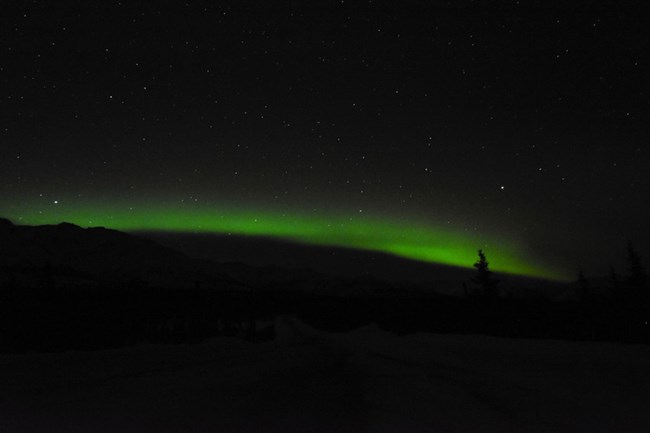The image depicts a mysterious night scene with a black, star-speckled sky. On the horizon, there's a gradual transition from a deep black to a faint grayish tint, with a striking green glow at the skyline. This green light, possibly from the setting sun or another source, radiates upwards, gradually blending into the dark sky. The foreground features the silhouette of a hilly terrain that slopes downwards to the right, while a valley rests at the base drenched in shadow. Within the dark terrain, faint silhouettes of trees, including identifiable pine trees on the right, are backlit by the eerie green glow. The whole scene carries a sense of serene and otherworldly darkness, interrupted only by that ethereal streak of green.